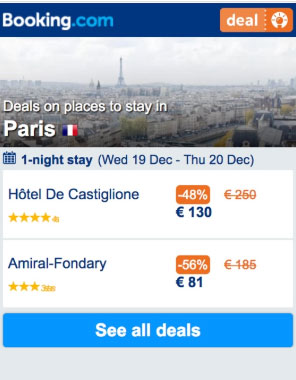This is a screenshot of the mobile version of the Booking.com website. In the top left-hand corner, the logo is prominently displayed with 'Booking' in white and '.com' in aqua blue against a blue urban-themed background. On the top right-hand side, there's an orange rectangle featuring a special offer icon of a light bulb and the text "Deals on places to stay in Paris" accompanied by a small French flag beside the word "Paris." Below this, details of a single-night stay from Wednesday, December 19th to Thursday, December 20th are provided, highlighted by a small calendar icon.

The first listed hotel is "Hotel de Castiglione," which boasts a 4-star rating. It's currently priced at €130, a significant reduction (48% off) from its original price of €250, shown crossed out. The second hotel listed is "Admiral Fondari," holding a 3-star rating. It is currently available for €81, offering a substantial discount of 56% off its usual price of €185.

At the bottom of the screen, there's a blue rectangular button labeled "See all deals," encouraging viewers to explore more options. The background behind the text "deals on places to stay in Paris" features a view of the Paris skyline under an overcast sky, adding a touch of local ambiance.